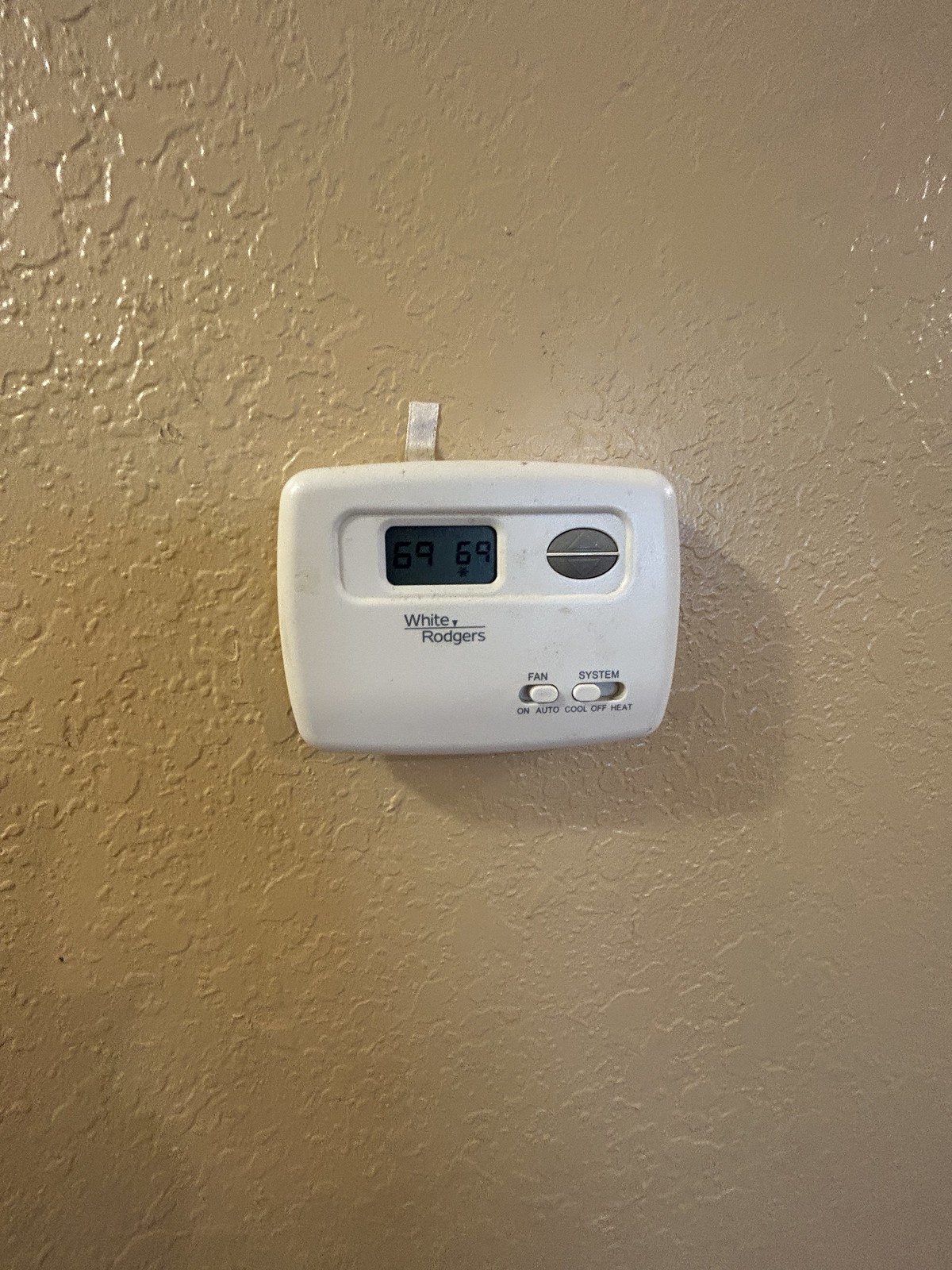The image features a detailed view of a wall thermostat affixed to a golden beige painted wall. The wall's textured patterns and designs subtly show through the paint, adding a layer of visual interest. The white thermostat, designed with a rectangular shape and rounded corners, prominently displays the brand name "White-Rodgers" in black lettering. The digital display on the thermostat indicates that the temperature setting is at 69 degrees Fahrenheit. In the lower right corner of the thermostat, two buttons are visible: the fan button, currently set to "Auto," and the system button, set to "Cool." The wall also captures a faint reflection of the thermostat, further emphasizing its presence in the image.